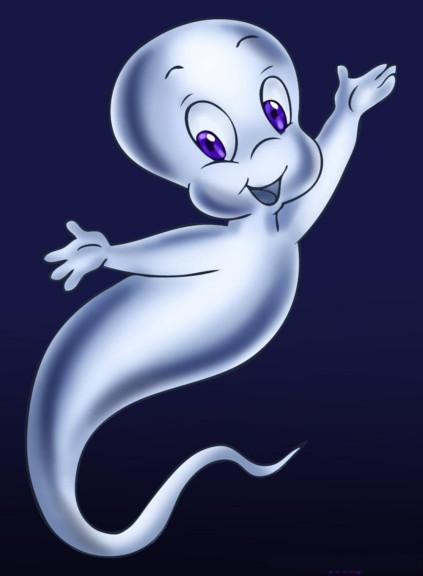The image features a portrait-oriented rectangle with a dark background composed primarily of a gradient that transitions from black in the bottom fourth to dark blue in the upper three-quarters. At the center of this background floats an animated ghost resembling Casper the Friendly Ghost. Casper has a silver-hued, slightly translucent body outlined in darker blue, making him stand out against the backdrop. He is facing the viewer with a cheerful expression, characterized by an open mouth, chubby cheeks, and large eyes with purple irises and black pupils. Casper’s body curves gracefully, with his tail curling from the lower left towards the center of the image. His arms are outstretched to his sides, each hand displaying four fingers. Casper is depicted without feet, giving the impression of mid-flight, and his overall demeanor is inviting and friendly.